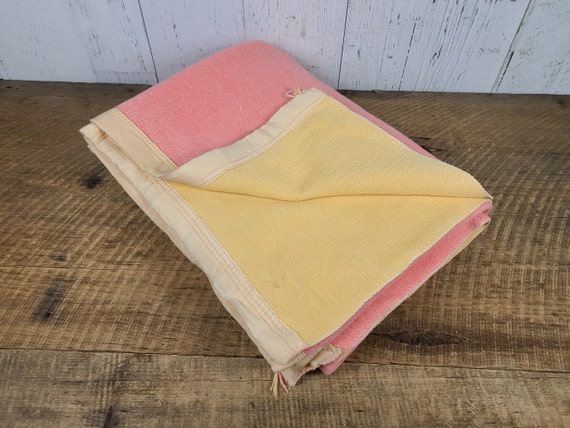This photo showcases a weathered, unfinished wooden flooring that meets the slightly faded white wood panels of a wall. Diagonally positioned from the top left to the lower right of the image is an old, stained reversible blanket. The blanket features a white satin border and is primarily salmon pink on the outer side, with a corner folded back to reveal the underside in a canary yellow shade. The blanket appears to be slightly dirty and shares the rustic aesthetic of its surroundings.